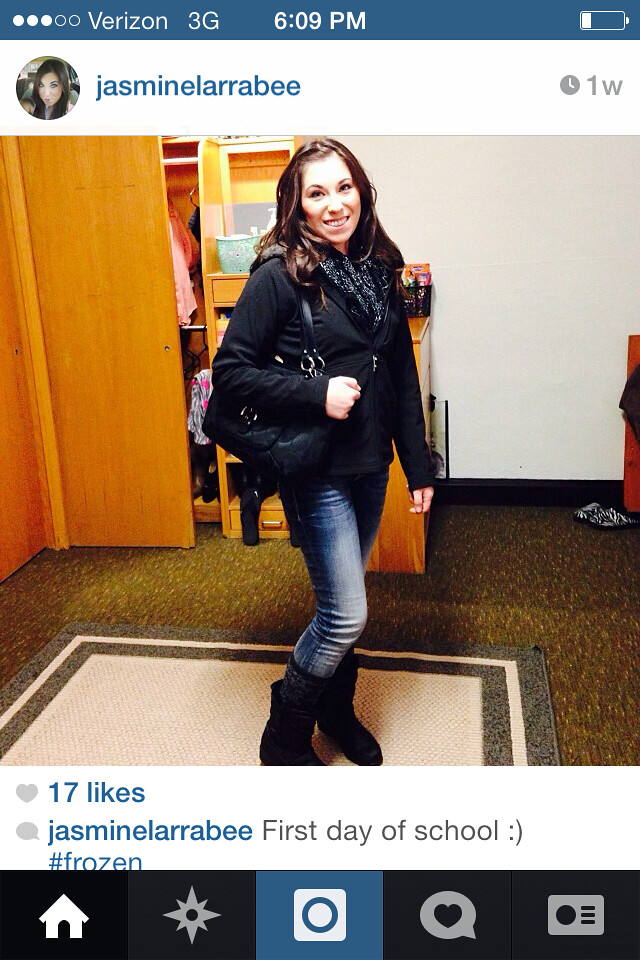In this image, we see a young woman named Jasmine Larabi, captured in a screenshot from her Instagram page on an old iPhone with Verizon 3G service at 6:09 p.m., and her battery is a quarter full. The photograph, posted a week ago and has garnered 17 likes, shows Jasmine standing on a rectangular rug with a brown border and a light tan center, in what appears to be her home.

Jasmine is dressed in a pair of blue jeans and black boots. She is wearing a black jacket, which appears puffy around the sleeves, along with a scarf around her neck. Draped over her shoulder is a black purse. Her dark brown hair is gently pulled back at the top and cascades down in soft curls framing her oval-shaped face. She is looking directly at the camera, smiling brightly.

Behind her, there is a partially opened closet with an orange door, built-in shelves, and a small counter, possibly situated in a corner of her apartment. The screenshot includes Instagram interface elements such as home and navigation buttons, post button, likes button, and news button, along with Jasmine's caption, "First Day of School :) #Frozen."